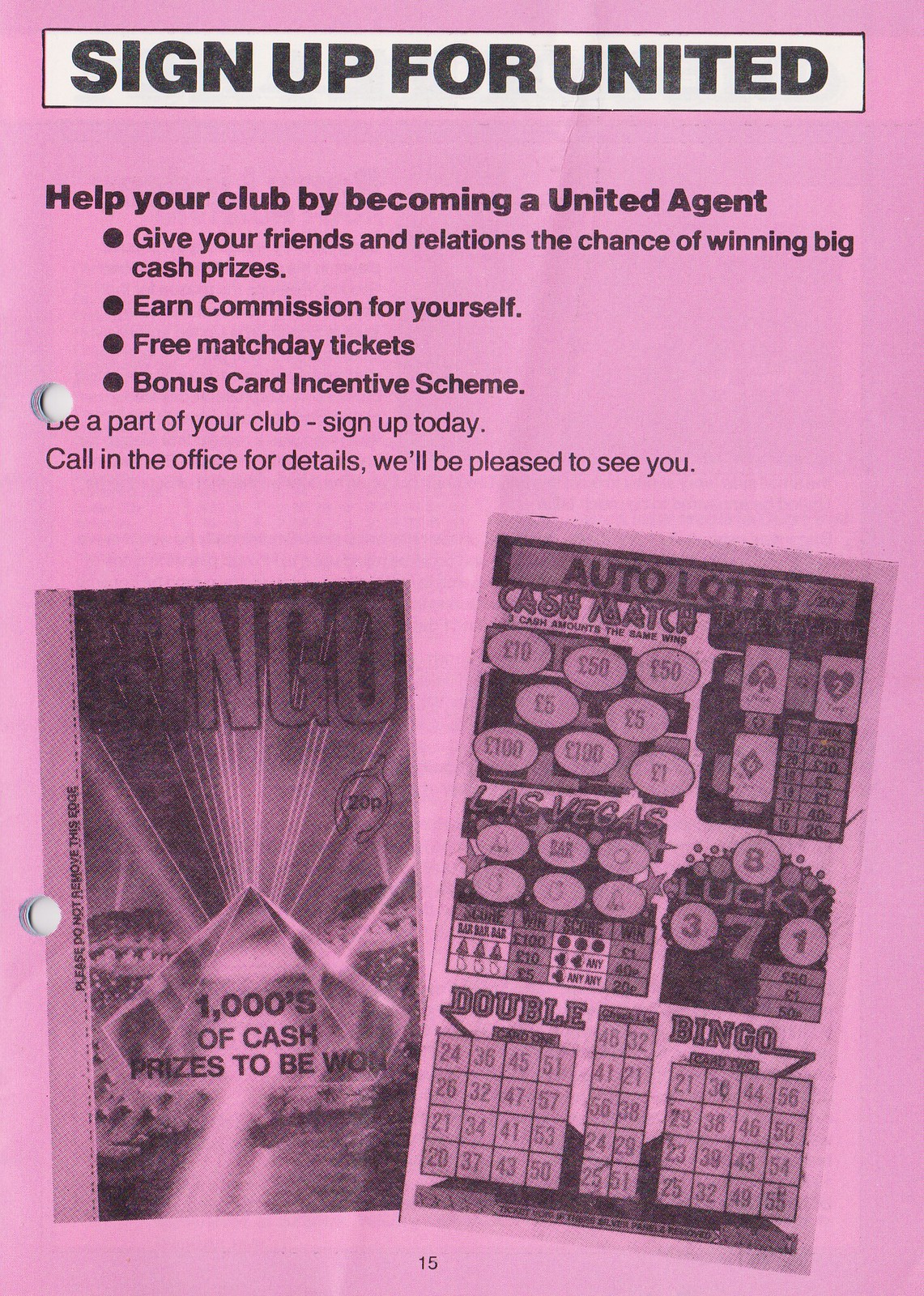The advertisement poster has a light purple and pink background, with two punch holes on the left side for binder storage. At the top, against a white rectangle, bold black lettering announces, "Sign up for United." Below that, in similar black text, it reads, "Help your club by becoming a United agent." The poster lists enticing benefits in black lettering with bullet points: 
 
- Give your friends and relations the chance of winning big cash prizes
- Earn commission for yourself
- Free match day tickets
- Bonus card incentive scheme

Further down, smaller black letters encourage, "Be part of your club, sign up today," and invite interested individuals to "call in the office for details, we'll be pleased to see you."

On the bottom left, there is a photo showcasing a lottery card with the word "Bingo" and white rating lines. Adjacent to it is a diamond-shaped feature that declares, "Thousands of cash prizes to be won." On the right side of the poster is an image of another lottery card labeled "Auto Lotto," presenting various numbers and the phrase "Double Bingo" at the bottom.